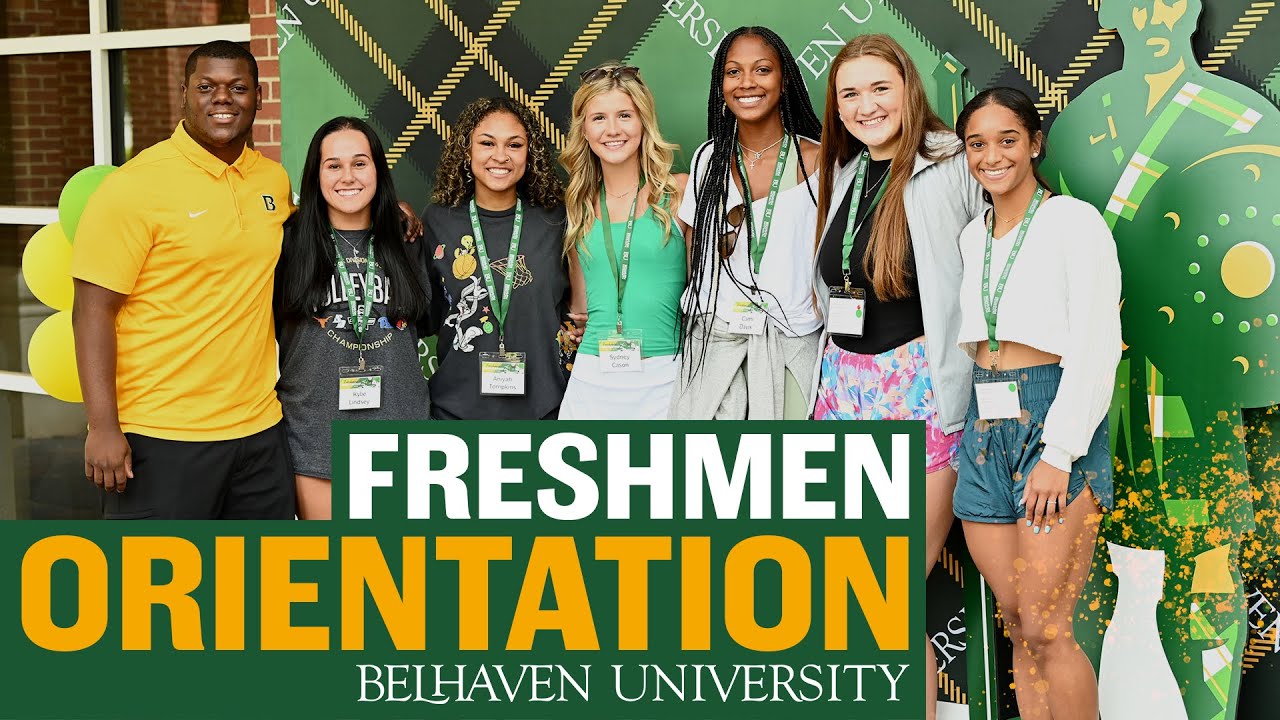The image depicts a vibrant and diverse group of seven university students lined up in front of a green, gold, and white plaid-themed backdrop at a freshman orientation event for Belhaven University. Prominently positioned on the backdrop, the text reads "FRESHMAN ORIENTATION" in large white and gold letters with "Belhaven University" inscribed in a unique font. The background features a striking cut-out of a green Scottish warrior holding a shield. Among the group, all wearing green lanyards with name tags, stands a tall man on the left in a bright yellow shirt, while the remaining six women are dressed in various shades of green, pink, black, orange, and white. All are smiling warmly, seemingly poised to welcome new students. The event exudes a spirit of giving and inclusivity, with an emphasis on community and school pride.